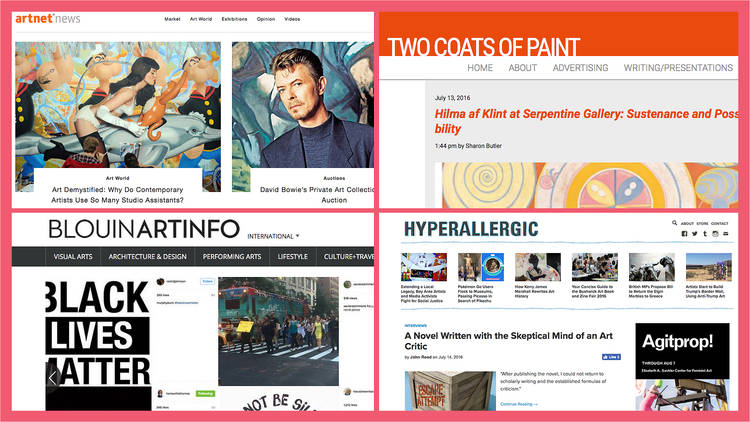The image depicts a detailed comparison of two website screenshots set against a salmon pink background. On the left screenshot, the website is titled "ArtNet News" with "ArtNet" in orange text and "News" in gray text positioned in the upper left-hand corner. The header section of the page lists five categories from left to right: "Market," "Art World," "Exhibition," "Opinion," and an illegible fifth category. Below the header, there are two images each accompanied by descriptive titles. The first image features a girl in white lingerie with black hair, riding a gray dolphin alongside sailor men figures. The title beneath this image reads, "Art World Art Demystified: Why Do Contemporary Artists Use So Many Studio Assistants?" in black text on a white background. The second image shows a man with brown hair and pale European features, standing in front of blue-colored artwork, wearing a dark blue denim shirt. The section below the image highlights "David Bowie's Private Art Collection Auction," followed by text categories "Visual Arts," "Architecture and Design," "Performing Arts," "Lifestyle," and "Culture and Travel."

The right screenshot showcases another website titled "Two Coats of Paint" in orange at the top, followed by a header and a paragraph heading "Hilma af Klint at Serpentine Gallery." Below this, there are more sections and pictures, including a section titled "Hyperallergic." Upon closer inspection, it becomes clear that there are actually four divided sections in this screenshot, contrary to the initial perception of two sections.